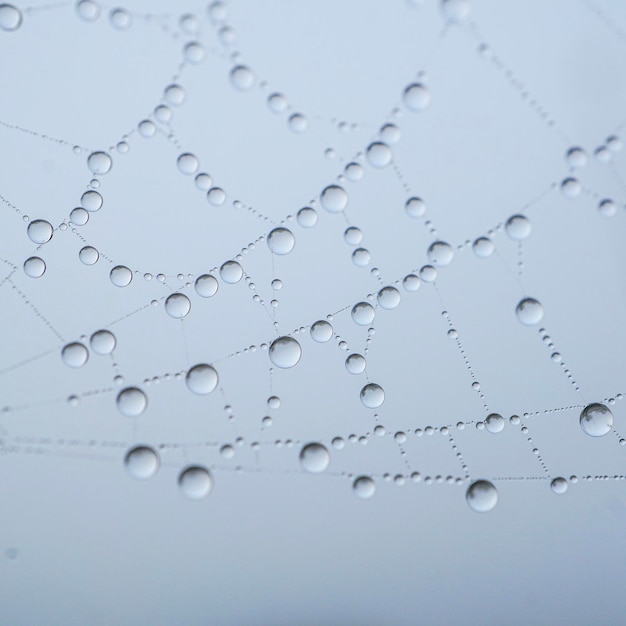The image showcases a light bluish gray background, uniformly dotted with perfectly round water droplets that vary in size. These droplets, appearing as raindrops, are meticulously distributed, creating a delicate and intricate lattice-like pattern reminiscent of a spider web. The larger droplets anchor the structure while the smaller droplets connect them in fine lines, enhancing the web-like appearance. The pattern, though somewhat scattered, suggests a natural, unplanned formation. The droplets appear as if suspended on the web, capturing a moment of stillness. The effect is a mesmerizing spectacle, transforming an ordinary spider web into a captivating and almost ethereal network of shimmering droplets against the pale background.